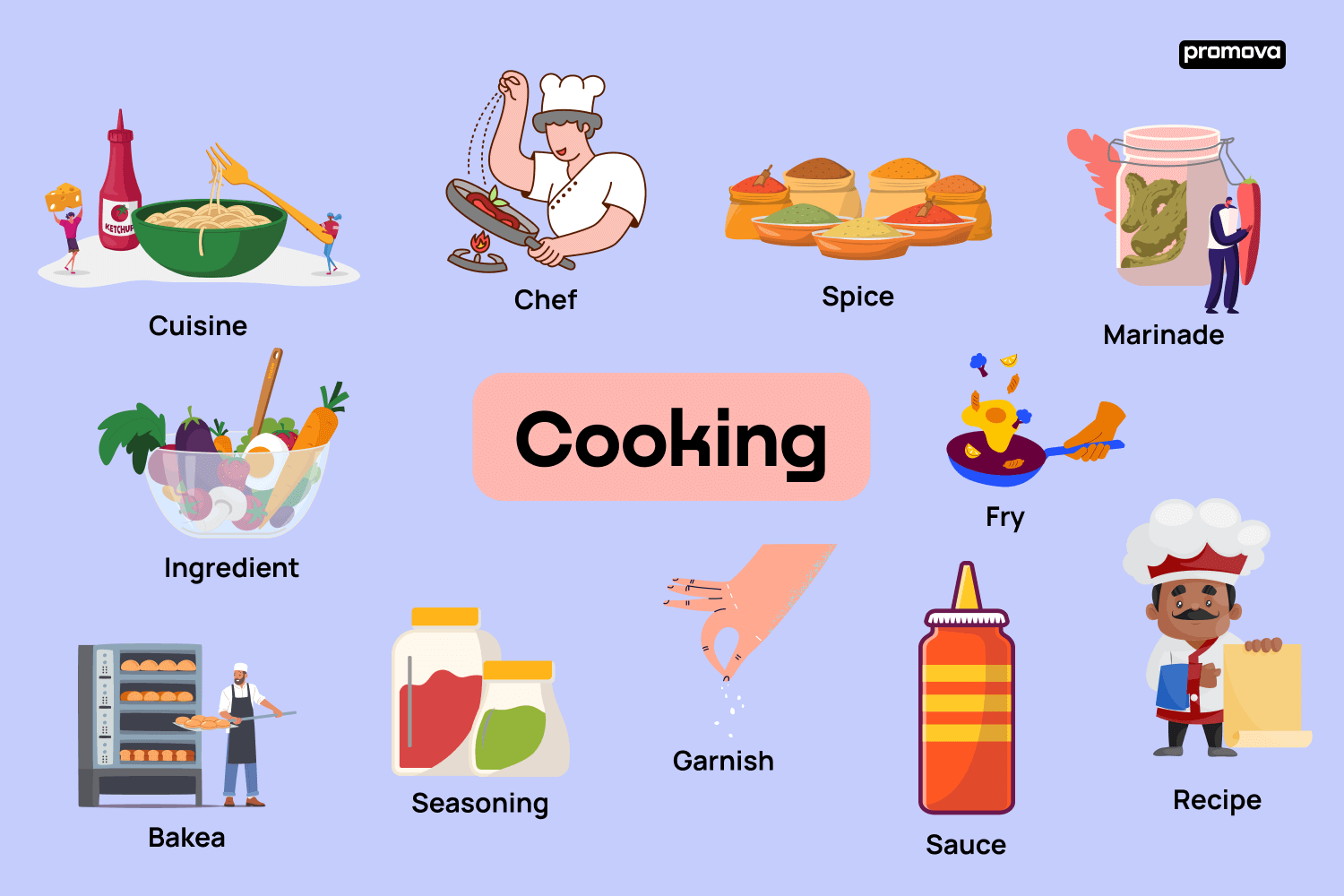The image features a light purple background with a central peach rectangle, bordered by rounded corners. At the center of the rectangle, the word "Cooking" is prominently displayed in black text. Surrounding this central title are a series of illustrated icons each labeled with terms related to cooking, each with detailed imagery. 

At the top-left corner, a label reads "Cuisine," accompanied by tiny characters in a bowl of spaghetti. To the right, a "Chef" illustration depicts a chef with a white hat and grey hair sprinkling something onto a skillet. Next is "Spice," represented by brown bowls of various spices. "Marinade" is illustrated with a man holding a large pepper, with a jar of pickles in the background.

In the middle row, to the left, an "Ingredients" label features a bowl of vegetables, and to the right, "Fry" is depicted with an egg frying in a skillet. "Recipe" is shown with a chef holding a scroll, while "Sauce" showcases a bottle colored white, red, and orange. "Garnish" has an illustration of someone pinching spice between their thumb and forefinger. "Seasoning" shows two jars, one red and one green, both with yellow lids. "Bake" (incorrectly labeled "Bakea") displays a man near an oven, seemingly making a brick oven pizza.

The bright and diverse color palette includes shades of black, white, gray, orange, brown, red, green, purple, pink, and yellow. The overall style is an artistic illustration emphasizing various facets of cooking through vibrant, detailed drawings.